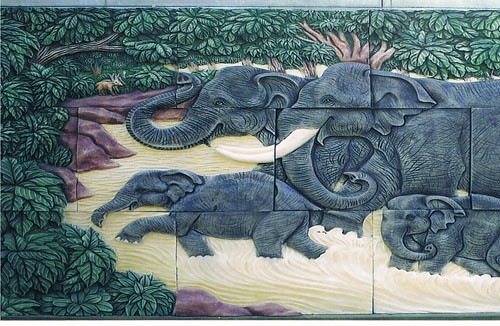The image features a richly detailed mural painted on a brick wall, depicting two adult elephants and two baby elephants in a naturalistic setting. The mural, which appears to be textured either through intricate painting techniques or a mosaic overlay, shows the elephants walking in a stream. The two adult elephants are positioned centrally and to the right, side by side, with one prominently displaying large tusks. The baby elephants are in the foreground; one is extending its left foot towards the edge of the stream, while the other has its trunk curved down into the water.

The mural captures a dynamic scene with a backdrop of green foliage, including small shrubs and leaves that border the upper and left sides of the image. Adding to the natural setting, grayish-brown rocks can be seen among the greenery. The stream water in the mural is rendered in tan or yellow hues, flowing over a sandy bottom with visible waves and lines, creating a cohesive, immersive portrayal of the elephants' habitat. The overall color palette includes tan, creamy, and dark gray tones, adding to the mural's lifelike appearance.